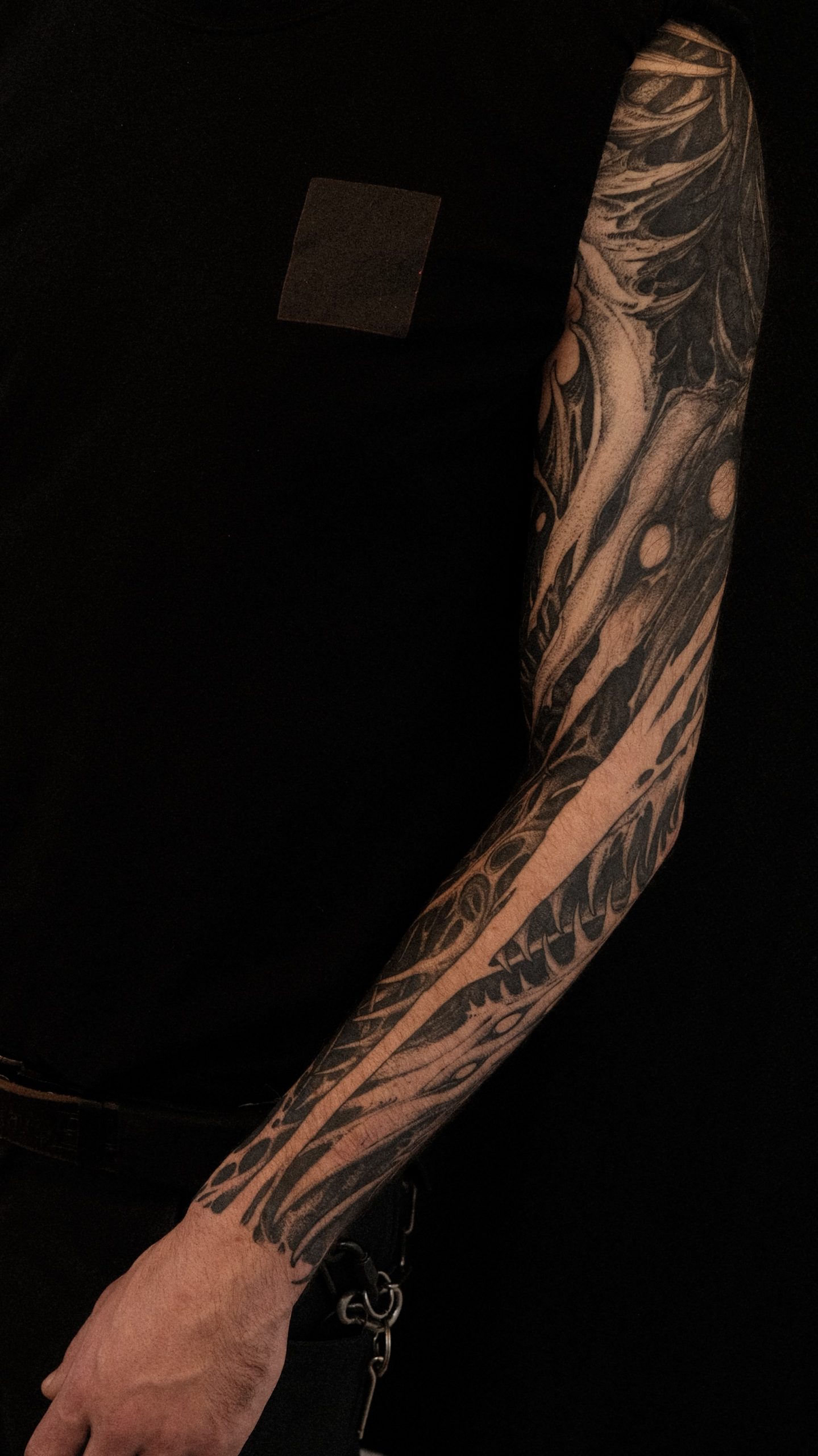The image features a close-up of a man's fully tattooed left arm, which stands out against a black background, further accentuated by his black shirt and black pants. The arm is adorned with a full-sleeve tattoo rendered in intricate black line work, creating a stark and impressive contrast. The tattoo covers the entire arm, starting from a clean line at the wrist and extending up to the shoulder. The design appears to be a chaotic yet mesmerizing mix of jagged, craggly elements resembling rotting wood, thorns, eyes peeking through, and possibly hinting at skeletal forms or faces, lending a gothic and somewhat spooky vibe. A small gray square is visible on his shirt, and a silver key ring with keys hangs from his belt loop, adding subtle details to his alternative aesthetic. The detailed, swirling designs suggest an immense amount of work and creativity, indicative of the man's unique lifestyle.